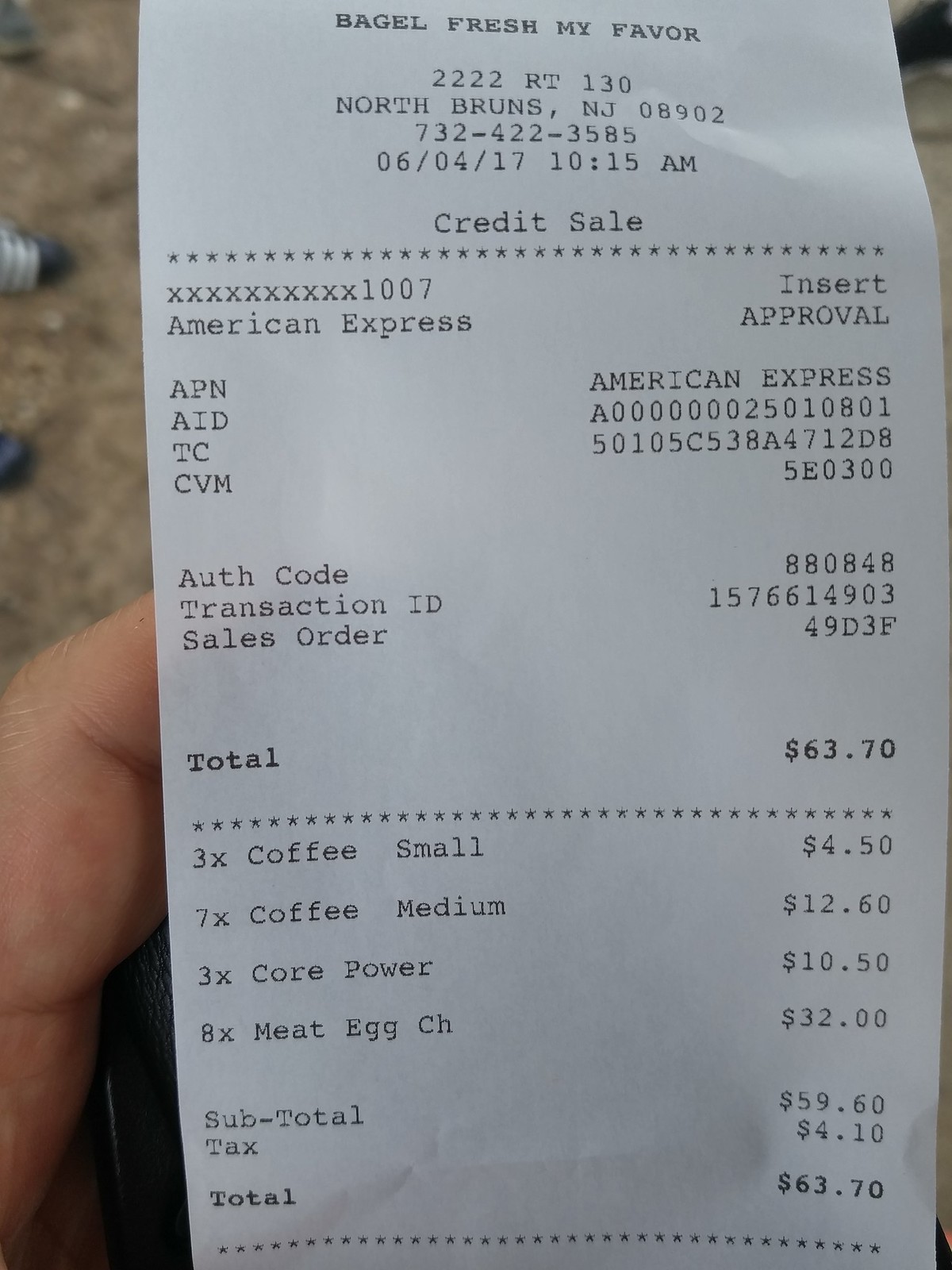A hand is holding a receipt from Bagel Fresh, a favorite eatery located in North Brunswick, New Jersey. The receipt is dated June 4th, 2017, with a timestamp of 10:15 AM. Bagel Fresh’s phone number is also visible on the printout. The purchase, totaling $63.70, was made using an American Express credit card. The itemized list includes three small coffees, seven medium coffees, three units of "Core Power" (details unspecified), and eight meat, egg, and cheese breakfast sandwiches. The subtotal came to $59.60, with an additional $4.10 in tax to reach the final amount. In the blurred background behind the hand, an indistinct surface is visible.